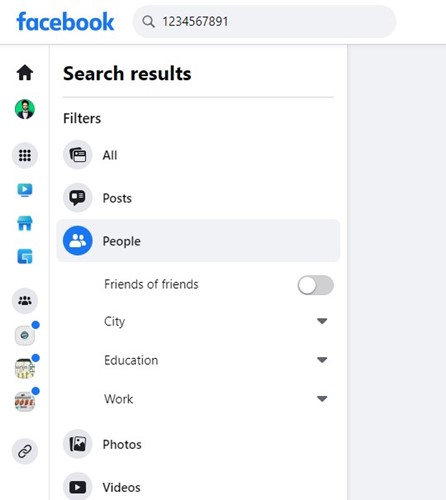In this image, reminiscent of a Facebook mobile website interface, the top left corner prominently displays the "Facebook" name in a bright blue color. Adjacent to it on the right is a search bar with the numbers "1234567891" entered in it. The search bar itself has a grayish background. Below the Facebook name, aligned vertically downwards, are several icons. The first is a home icon, followed by a profile picture icon depicting a person in a black and white shirt within a green circular frame. The subsequent icon is a circle composed of several smaller, darker circles forming a square shape. This is followed by three blue-colored icons: a play button, a shopping store symbol, and a square whose function is unclear. Below these, there are three additional icons, each marked with a blue circle on their top right corners. In the top middle section of the image, the words "Search Results" are displayed, with "Filters" situated below. Under the "Filters" heading, the categories "All," "Posts," "People," "Photos," and "Videos" are listed.